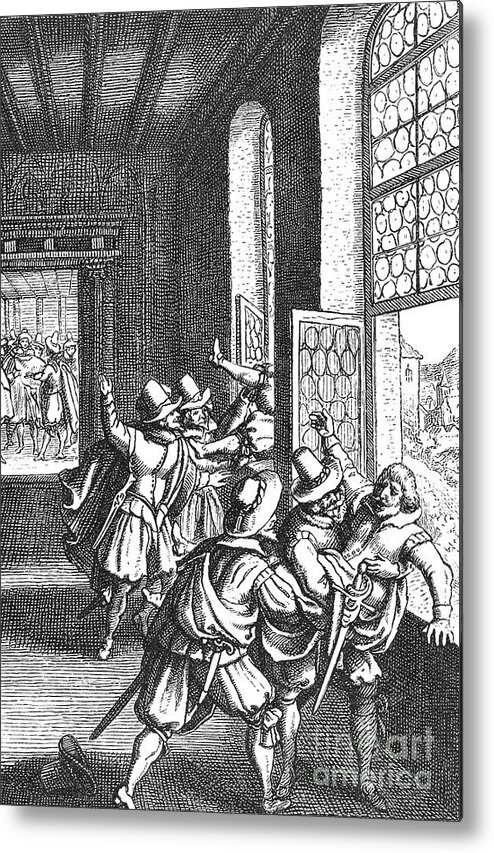This black and white print illustration, possibly a pencil drawing, depicts a tumultuous scene in a long hallway of what appears to be a castle or grand building, its architecture suggesting a period around the 1500s to 1700s. Wooden walls and ceilings frame the chaotic event, which is punctuated by light streaming through large, open windows on the right side. The distressed expressions of the men involved add to the drama. In the foreground, two groups of men, all donned in period-specific clothing—fluffy fabric outfits with shorter pants, pilgrim-style hats, and swords around their waists—are engaged in a fierce struggle. Each group is lifting a man, seemingly ready to push or throw him out of the open windows. The men's faces express extreme distress, especially those being threatened with defenestration. The background showcases another window with three men similarly poised to throw a fourth out. The recognizable detail of "Fine Art America" inscribed in the bottom right provides a clue to the artwork's reproduction source.